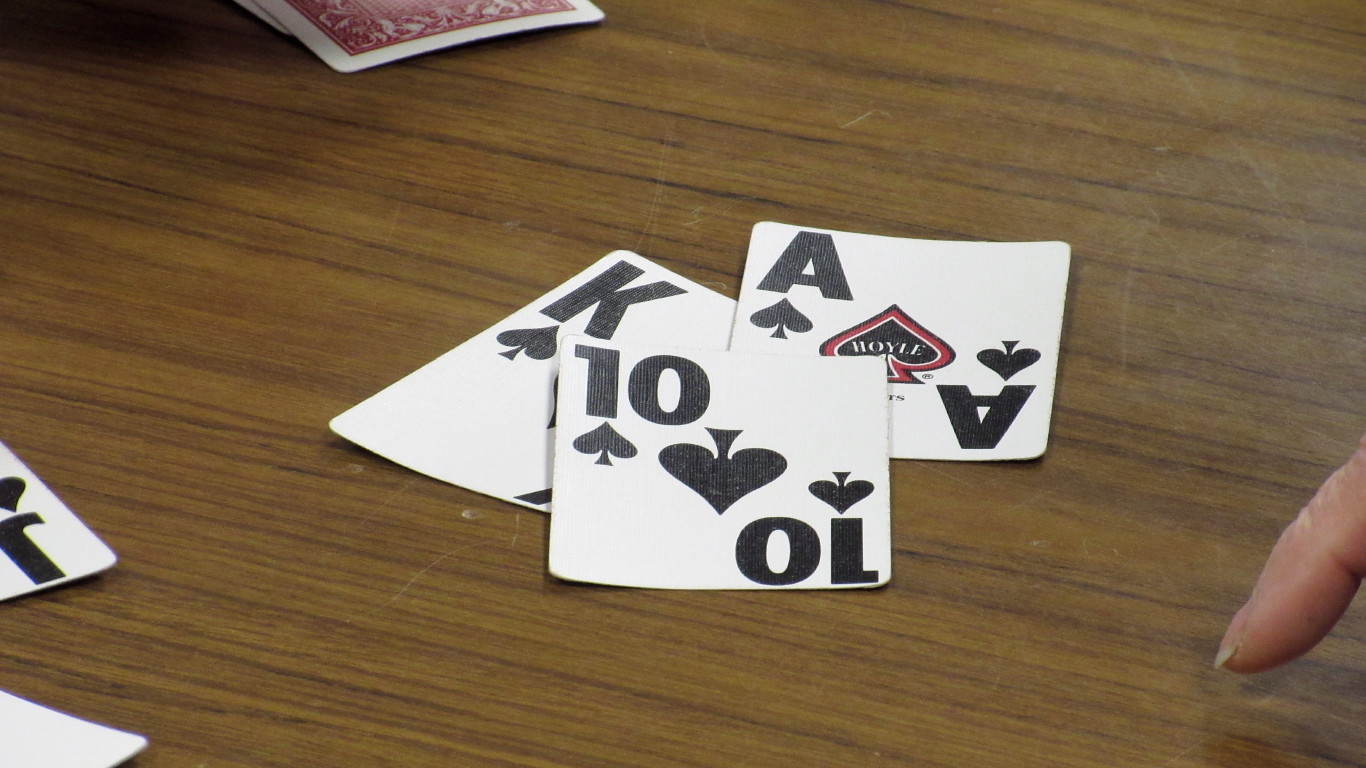The image features a close-up of a table with several playing cards arranged on it. On the bottom right, a fingernail is visible, indicating a person is pointing downward. The arrangement of the cards includes three cards prominently displayed in the center: a Jack of Spades on the left, an Ace of Spades in the middle which is distinguished by a unique red outline around the spade symbol, and a Ten of Spades on the right. In the background, at the top left, there are two cards facedown with a red decorative design on their backs. The focal point of the image is the central trio of playing cards, with the detailed spade designs providing a striking visual contrast.